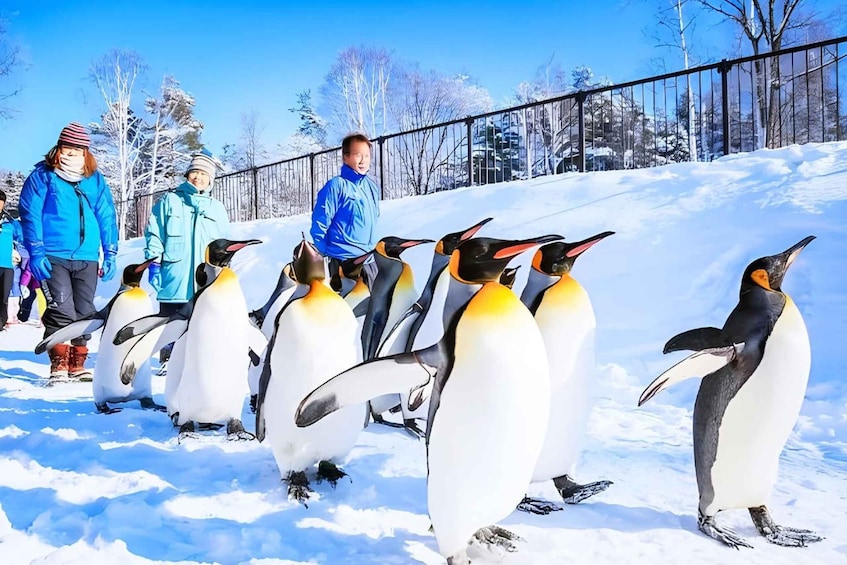This vibrant daytime photograph captures a group of about a dozen Emperor penguins confidently marching forward through a snowy landscape. The penguins, characterized by their white stomachs, yellow tops of the chest just beneath their heads, and orange-tinted beaks with black tips, feature distinctive black faces, backs, wings, and feet. Among them is a backdrop of crisp, clear blue sky and a snowy forest with trees dusted in white. To the side, a hilly incline rises, topped with a metal gate designed to be just high enough to contain the penguins.

Several people, potentially visitors or handlers, follow behind the penguins. Two women and one man can be noted, all clad in winter attire comprising variously shaded blue puffy jackets and scarves. The man is distinguishable by his striking red boots. Additionally, two of the individuals are wearing winter hats. The sunlight, coming from the top right corner of the image, casts vivid shadows across the entire scene, contributing to the overall brightness and clarity of the composition.